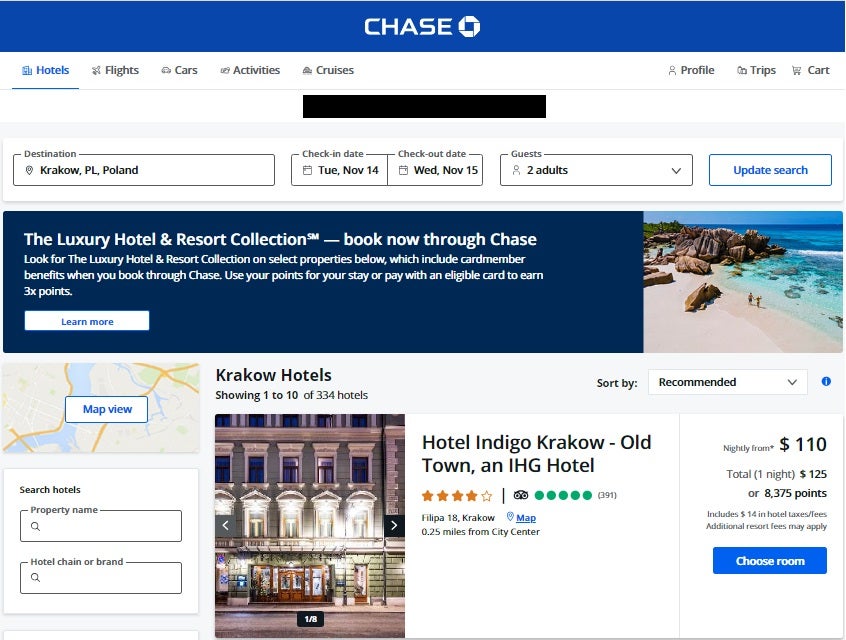The image captures a detailed interface of a Chase travel booking app, where users can plan their trips with various options including hotels, flights, cars, activities, and cruises. The app interface features a modern, clean design with the "Hotels" tab highlighted in blue along the top, while the others—flights, cars, activities, and cruises—are gray.

On the top right, the app provides links to "Profile," "Trips," and "Cart." The central section of the page appears to be blacked out for privacy, potentially concealing sensitive information such as an account number. Within this section, users can enter details for their travel plans, including: 

- **Destination:** Krakow, Poland
- **Check-in Date:** Tuesday, November 14th
- **Check-out Date:** Wednesday, November 15th
- **Guests:** Two adults

A prominent "Update Search" button in blue is positioned to the right.

Below this, a stunning visual element captures attention—a large banner photograph of a picturesque coastal scene taken from about 80 feet in the air, featuring azure waters, slight waves, and uniquely shaped, prehistoric rock formations. This inviting image serves as a backdrop to highlight the luxury hotel and resort collection available through Chase. It reads:

"The Luxury Hotel and Resort Collection. Book now through Chase. 
Book for the luxury hotel and resort collection on selected properties below, which include card member benefits when you book through Chase. Use your points before you stay or pay with an eligible card to earn three times points." Accompanied by a "Learn More" button on the dark blue background.

Further down, the app transitions to a map view interface with search fields for "Hotels," "Property Name," or "Hotel Chain or Brand." It displays a list of hotels in Krakow, starting with the first entry:

- **Hotel Name:** Hotel Indigo Krakow Old Town, an IHG Hotel
- **Rating:** Four stars out of five
- **Reviews:** Five green circles, likely from TripAdvisor
- **Address:** Philippa 18, Krakow, 0.25 miles from the city center
- **Rate:** From $110 per night, total of $125 for one night or 8,375 points, which includes $14 in hotel taxes and fees. 
- **Additional Info:** Additional resort fees may apply
- **Action Button:** "Choose Room"

The hotel is depicted with a night-time photograph showcasing its neoclassical stone architecture, adorned with wooden doors and a greenish facade. It is noted as image one out of eight available for the user to view. The interface is intuitive, encouraging users to explore and book hotel options effortlessly.